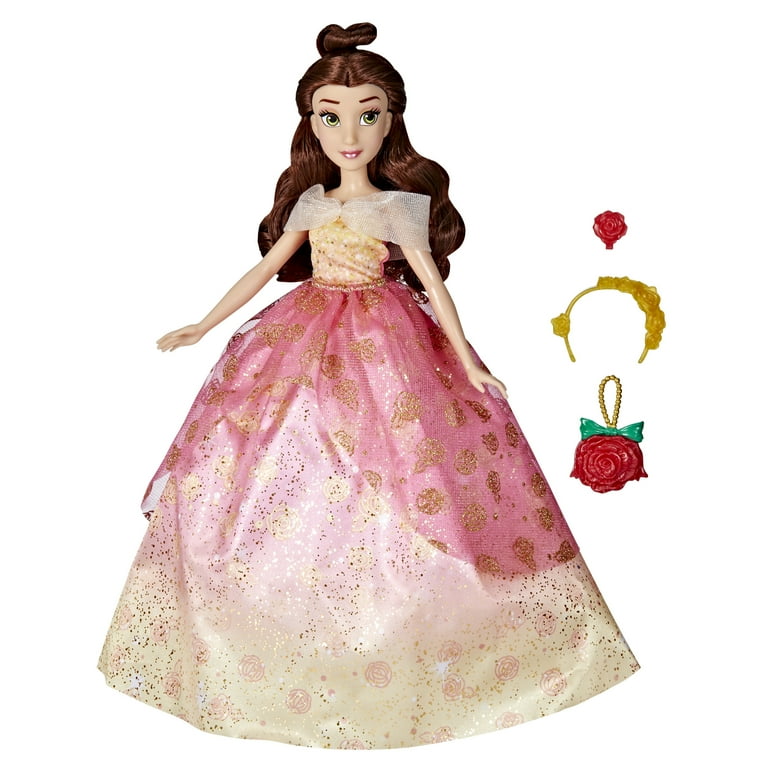This image features a princess doll with long, wavy, dark brown hair styled in an updo knot atop her head while the rest of her hair cascades down to her shoulders. She has striking, large yellow-green eyes with black pupils and white accents, complemented by reddish lipstick on her lips. The doll is dressed in an elaborate princess gown characterized by its poofy nature and layers that conceal her legs entirely. The upper part of the dress includes slightly transparent white fabric covering her shoulders, while the main body of the dress boasts a mix of yellows and pinks, adorned with golden flower patterns and dark orange sparkles. Her arms are slightly extended outwards. To the right of the doll, there are three shiny accessories which include: a red rose, a yellow headband adorned with yellow roses, and a larger red rose with a green bow that hangs from a silver ball chain, likely intended to embellish the doll further.